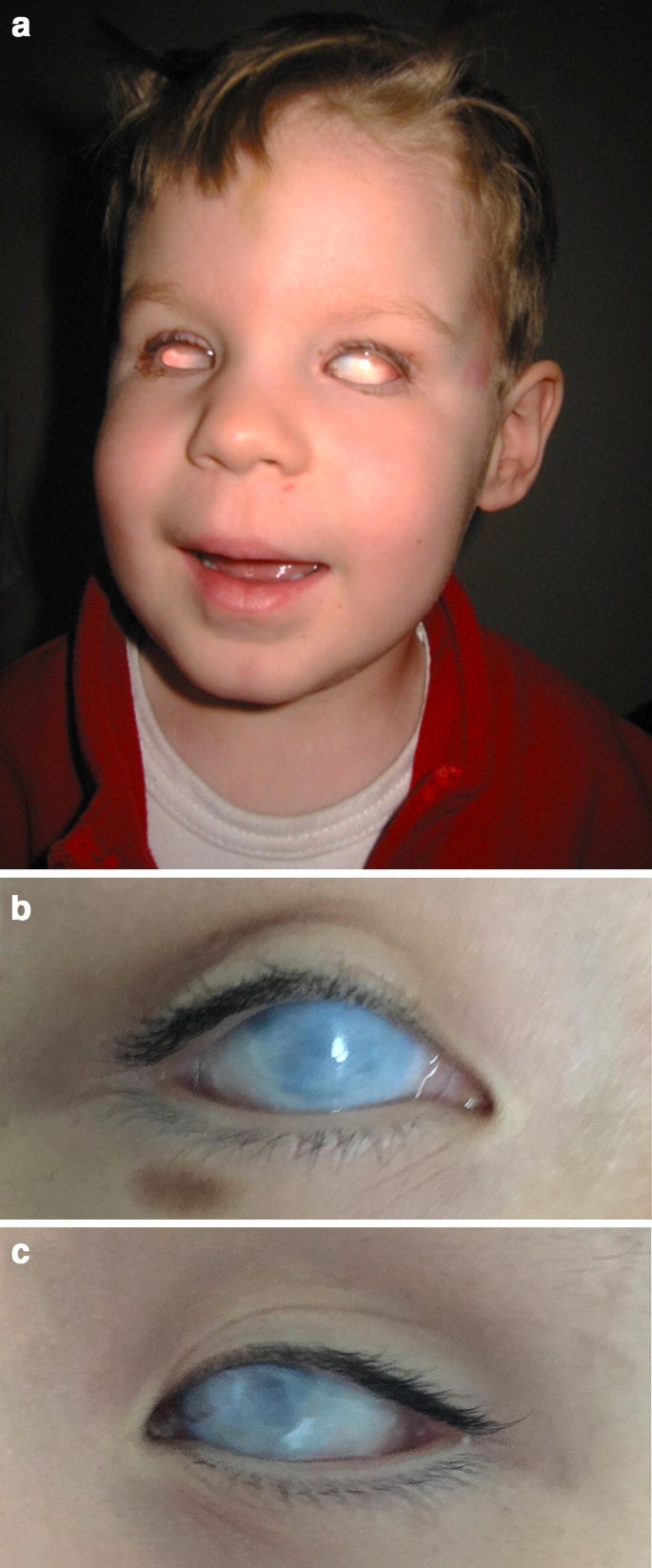This image presents a poignant view of a young boy, likely around four years old, with sandy blonde hair and dressed in a red jacket over a white t-shirt. The photograph is divided into three labeled sections: A, B, and C. Section A features a full view of the child, whose eyes are strikingly unusual. Both eyes exhibit a significant white, glossy covering, suggesting a severe ocular condition. The otherwise bright blue irises are barely visible beneath this cloudy layer, giving a disconcerting impression that his pupils are missing.

Sections B and C provide detailed close-ups of the boy's right and left eyes, respectively. In these up-close shots, one can discern more clearly the underlying structure of the eyes, including the pupils and irises, which appear to be masked by a pale, jelly-like layer. His right eye (B) reveals a slight bruise or birthmark beneath the lower eyelash, while the left eye (C) seems to turn inward slightly, creating a subtle cross-eyed effect. This arrangement and outlook suggest that the child might be suffering from a serious eye condition, potentially obscuring his vision. The underlying tone of the image is both distressing and empathetic, emphasizing the boy's sweet demeanor amidst his evident medical struggle.